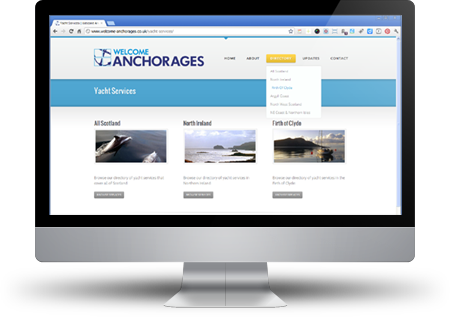The image is a computer-generated mock-up depicting what appears to be an iMac-like device, though it lacks the distinguishing Apple logo. Set against a white, transparent background, the mock-up casts a realistic shadow, drawing attention to its three-dimensional appearance. The screen showcases a web page dedicated to travel, albeit with blurred content due to the small image size, making specific details hard to discern. However, the visible text prominently includes "Welcome Anchorages," accompanied by an anchor logo. Adjacent to this is a drop-down menu. Below this section lies a sleek blue bar labeled "Yacht Services." The web page then transitions back to a white background, presenting information on three different locations: Scotland, Northern Ireland, and the Firth of Clyde—possibly indicating a peninsula. Each location is highlighted with corresponding images and a "more info" link.